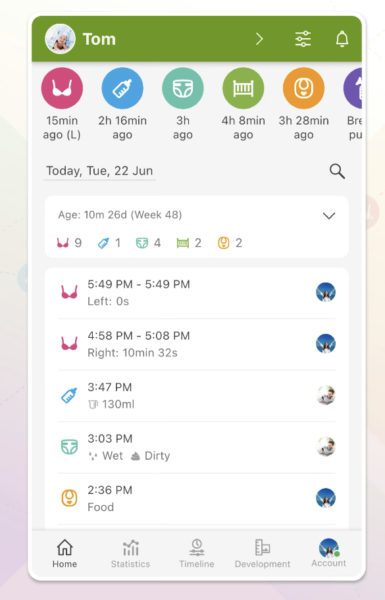This image depicts a detailed interface of a breastfeeding and baby care tracking app. The main screen shows records of breastfeeding sessions, indicating the times and durations of each session to help parents monitor their baby's feeding schedule. The app also appears to track additional information such as whether the milk was given directly or via a bottle, as well as diaper changes, noting whenever the baby has a bowel movement or urinates. 

The baby in the app is named Tom, whose age is specified as 10 months and 26 days, or week 48. Dominating the top of the screen is a green bar displaying "Tom" horizontally across it, possibly summarizing his current state or providing an overview of the tracked activities. The user interface includes a series of buttons at both the top and bottom for easy navigation and entry of new data points, ensuring comprehensive monitoring of the child’s daily routine and well-being.